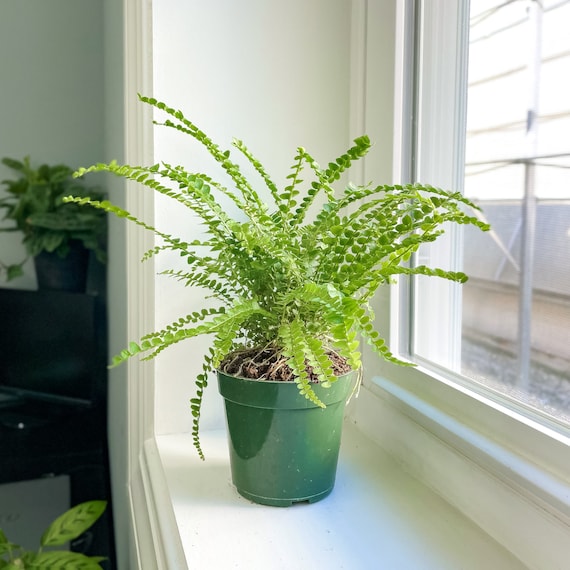This photograph captures the view from inside a house, focusing on a potted fern in a deep green plastic pot seated on a wide, white-painted windowsill. The fern, with its light green fronds elegantly arching upwards and outwards, commands the center of the image. To the right, the bright light filtering through a glass pane with a white frame highlights the neighboring building outside. In the background, there's another small potted plant resting atop what appears to be a bench or possibly a stand-up piano. Additionally, the bottom left corner reveals the green leaves of another plant situated on the ground, adding depth to the scene. The overall composition is an interplay of indoor greenery framed by the bright exterior light.